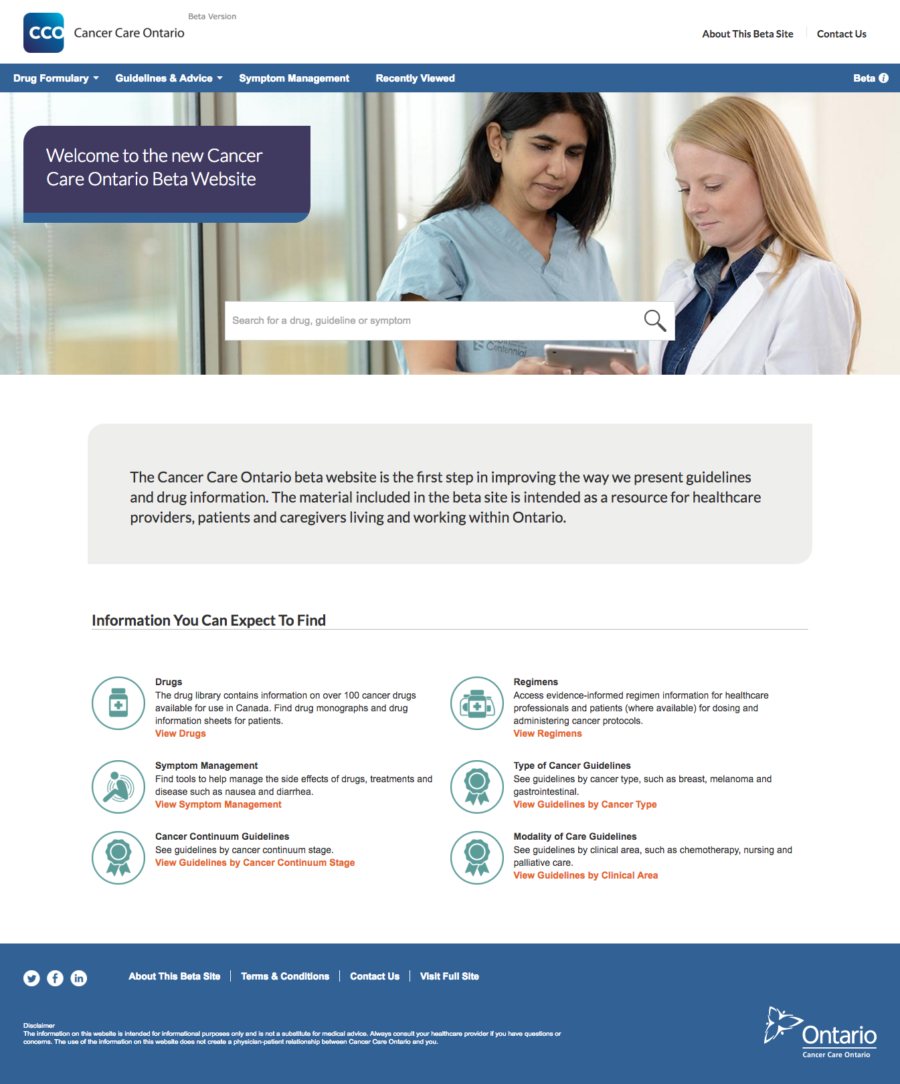This screenshot captures the homepage of the Cancer Care Ontario (CCO) beta website. At the top, within a teal box, the logo "CCO" is prominently displayed, accompanied by the text "Cancer Care Ontario" directly beneath. Above this site header, the option "Contact Us" is available. 

Below the header, within another teal rectangular box, various navigation options are listed: "Drug Formulary," "Guides and Advices," "Symptom Management," and "Recently Viewed." Positioned below these options is a welcoming image featuring two women, presumably a doctor and a nurse, with one writing a prescription. The overlay text on the image reads, "Welcome to the new Cancer Care Ontario beta website," alongside a search bar labeled, "Search for a drug, guideline, or symptom."

Further down, in a gray box, the website's purpose is elaborated: "The Cancer Care Ontario beta website is the first step in improving the way we present guidelines and drug information. The material included in the beta site is intended as a resource for healthcare providers, patients, and caregivers living and working within Ontario. You can expect to find drugs, symptom management, cancer continuation guidelines, regimens, type of cancer guidelines, modality of care guidelines."

At the bottom of the screenshot, a darker teal box features additional navigation options such as "Beta Site Terms and Conditions," "Contact Us," and "Visit Full Site." The Cancer Care Ontario logo, which includes a butterfly, appears prominently, reflecting the organization's identity.